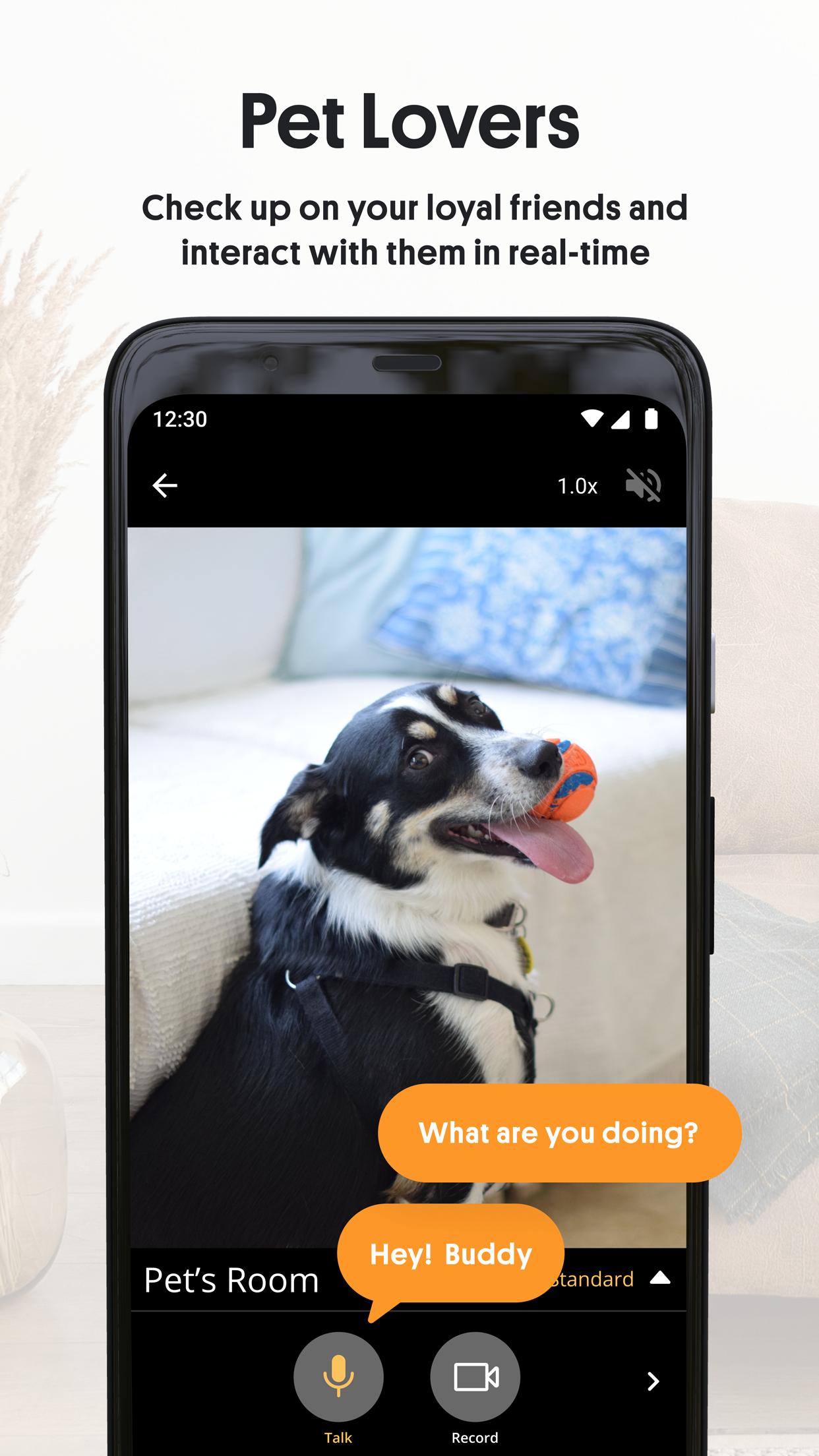The image depicts a mobile phone screen with a video call in progress. On the phone screen, there is a high-resolution image of a large black and white dog that closely resembles a collie. The dog is holding an orange tennis ball with blue stripes slightly off to the side of its mouth.

Starting at the top of the phone screen, the time is displayed in black as 12:30. To the right of the time, there is the Wi-Fi icon, an unidentified triangle icon, and a battery icon showing the current battery level.

On the next line, an arrow pointing to the left is situated on the left side, followed by ample black space. In the middle of this line, „1.0X” denotes the zoom level. To the right, a grayed-out speaker icon with a slash through it indicates that the speaker is muted.

The background of the video call shows a neatly made bed with a white bedspread. On the bed are two pillows: the one in the front has a darker blue floral pattern and the one behind it features a lighter blue pattern.

Superimposed on the dog's image, there are two orange text bars. The first bar, positioned across the top of the dog's image, reads "What are you doing?" The second bar, below it and styled as a thought bubble, states "Hey, buddy!" both written in a friendly, conversational tone.

At the bottom, the text "Pet's Room" is displayed in white, indicating either the label for the room or the name of the app in use. On the right side of the screen, a yellow microphone icon suggests that someone is talking to the dog. Adjacent to this is a video camera icon, representing the video call feature, and an arrow pointing right.